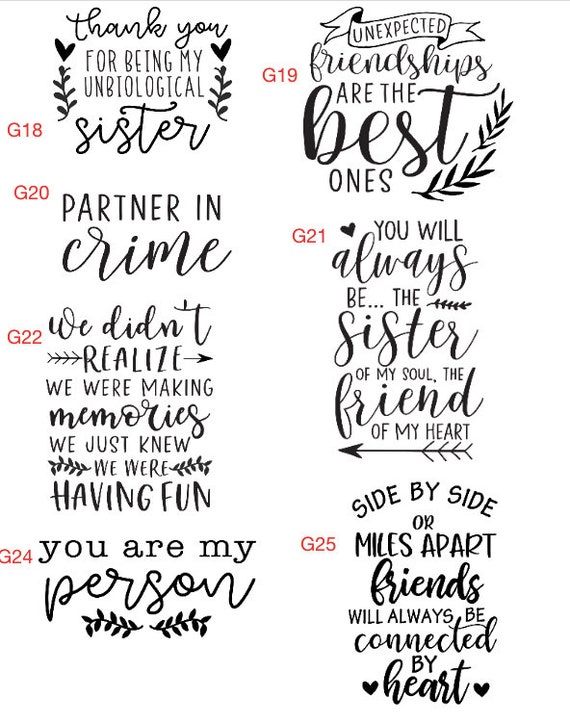This photograph features a collection of seven items numbered G18 through G25 (with G23 missing) that appear to be stickers, decals, or temporary tattoos, each showcasing handwritten phrases in black ink. Arranged in two columns—four on the left and three on the right—the phrases have a heartfelt and friendship-oriented theme, resembling sentiments found on greeting cards. The left column includes: "Thank you for being my unbiological sister," "Partner in crime," "We didn't realize we were making memories, we just knew we were having fun," and "You are my person." The right column features: "Unexpected friendships are the best ones," "You will always be the sister of my soul, the friend of my heart," and "Side-by-side or miles apart, friends will always be connected by heart."